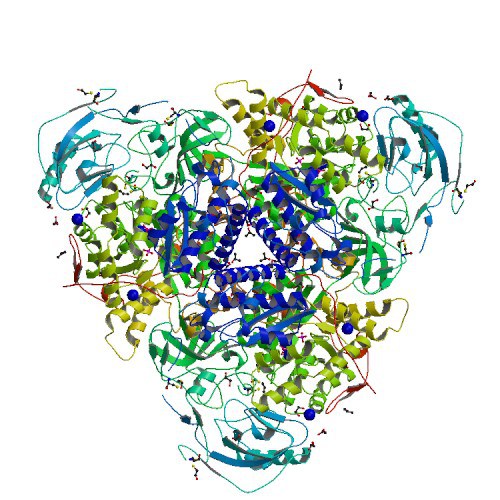The image features an upside-down triangular shape on a white background, filled with intricately interconnected squiggles of various colors. These squiggles have a multitude of hues, including royal blue, violet, teal blue, sky blue, brownish red, tan yellow, touches of pink, and orange. Some squiggles appear more like sausage curls or spiraled confetti, while others are straighter, resembling curly ribbons. All of these vibrant lines are connected by fine, hairline-thin lines, giving the appearance of being meticulously connected by strings. The overall image has an abstract quality, reminiscent of proteins or prions folding, with a transparent background that keeps the focus entirely on the colorful squiggles within the triangular form.